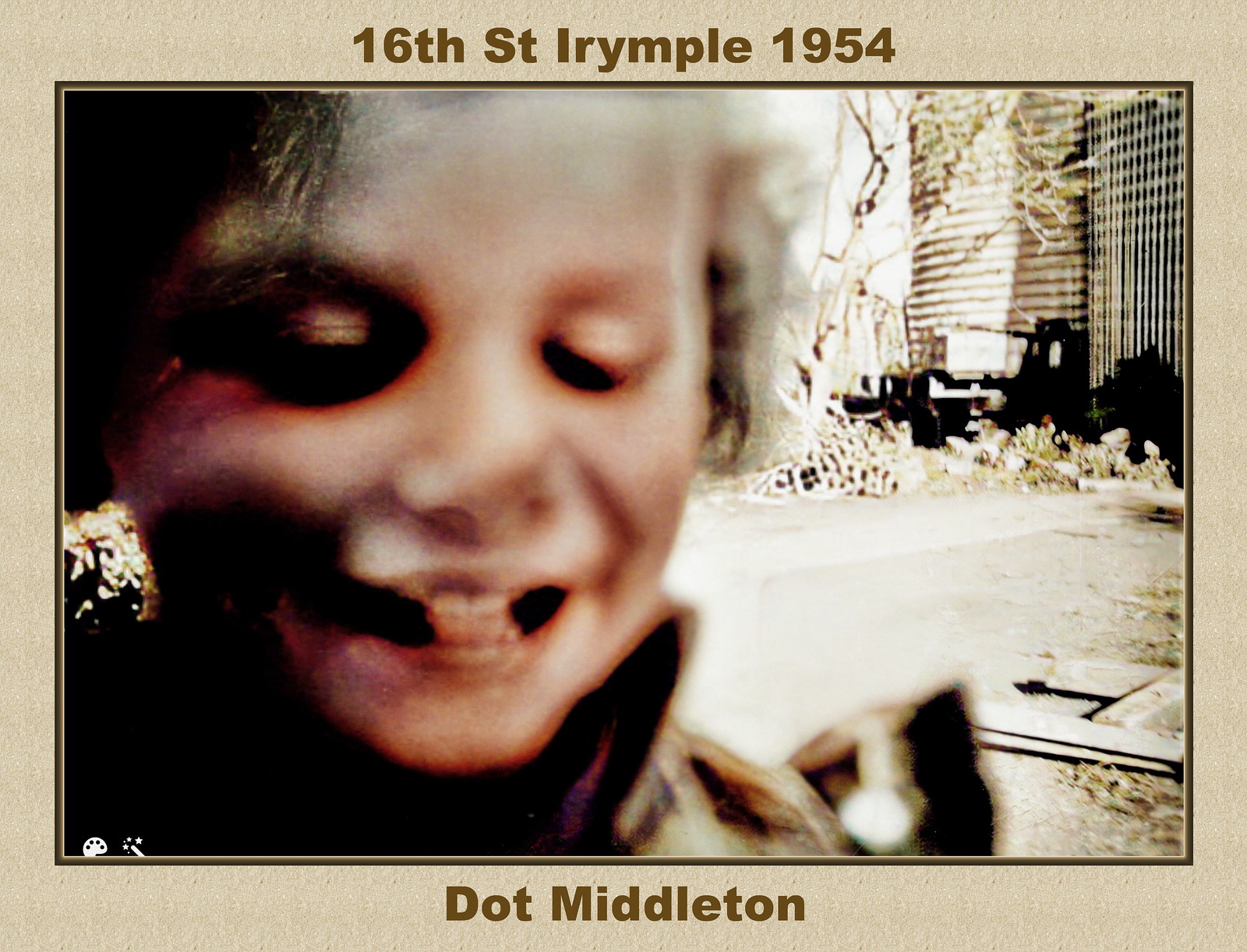This photograph, a wide rectangular image digitally framed, is presented on a textured light tan background with a thinner border on the left and right and thicker borders on the top and bottom, which have a dark greenish-brown inner color. At the top of the image, in bold greenish-brown font, it reads "16th Street, Iron Pole, 1954," while the bottom similarly states "Dot Middleton." The photo predominantly features a super zoomed-in, blurry face of a child positioned to the left, with some details indicating a possible white child with blonde hair and a few visible front teeth. The child's face is overexposed and discolored, blending into the aged, light brown toned photo. Off to the right, the background suggests an outdoor setting with a gray road, tall buildings, and tree silhouettes, all equally blurred and faded, enhancing the image's nostalgic, vintage feel.